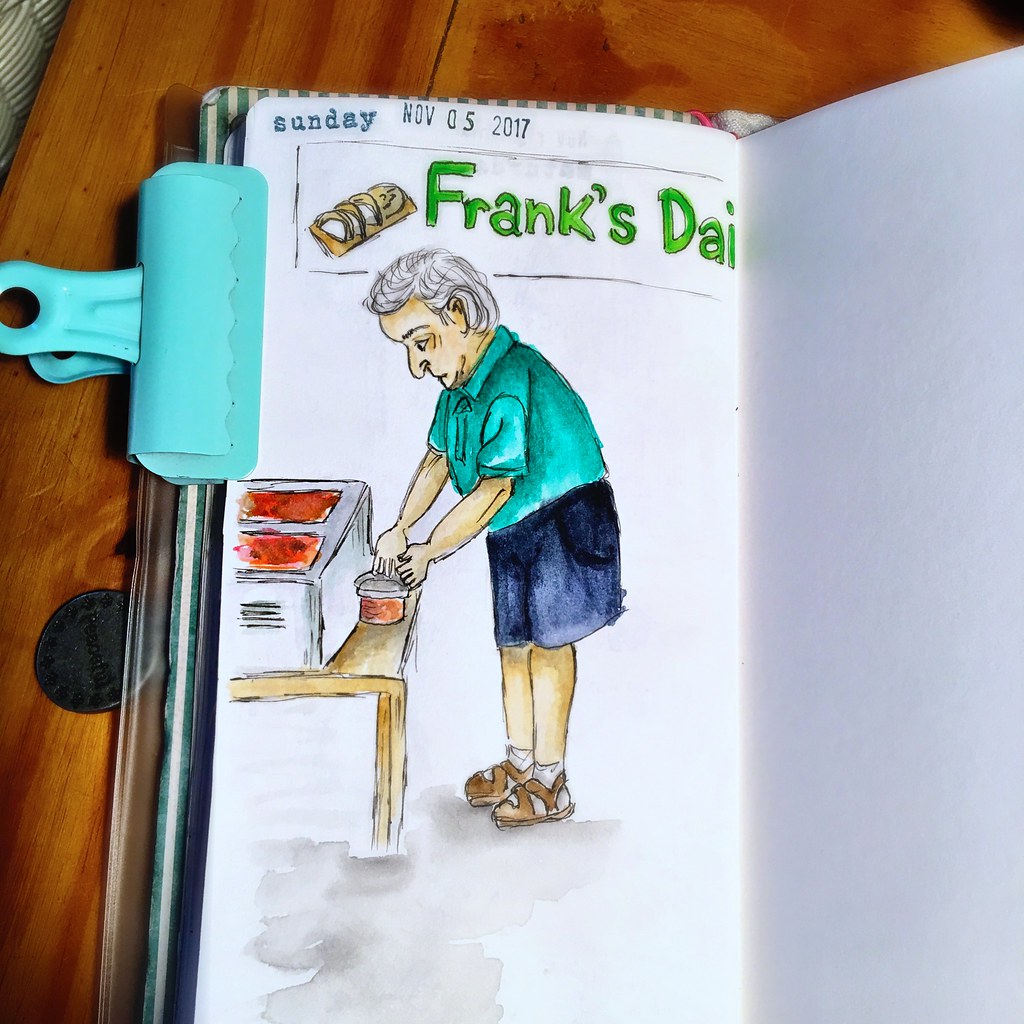The image is a detailed watercolor sketch of "Frank's Day" dated Sunday, November 5, 2017, within a small, striped green and white sketchbook. The sketchbook, lying open on a light brown wooden table with visible vertical boards, is held open by a turquoise bulldog clip at the top left-hand side. The drawing features an elderly man named Frank, with slightly long gray hair and light skin, dressed in a teal short-sleeved shirt, blue shorts, white socks, and brown Teva-style sandals. Frank is depicted looking down, seemingly in the act of preparing or handling some food. In front of him is a silver implement resembling toaster slots, and his hands rest on a circular object. The background also includes a visible coin on the table near the sketchbook. The page is topped with the words "Sunday" and "NOV 05 2017" stamped in ink, and the title "Frank's D.A.I" is written in a rectangular frame accompanied by an icon resembling coconut pieces on a platter.